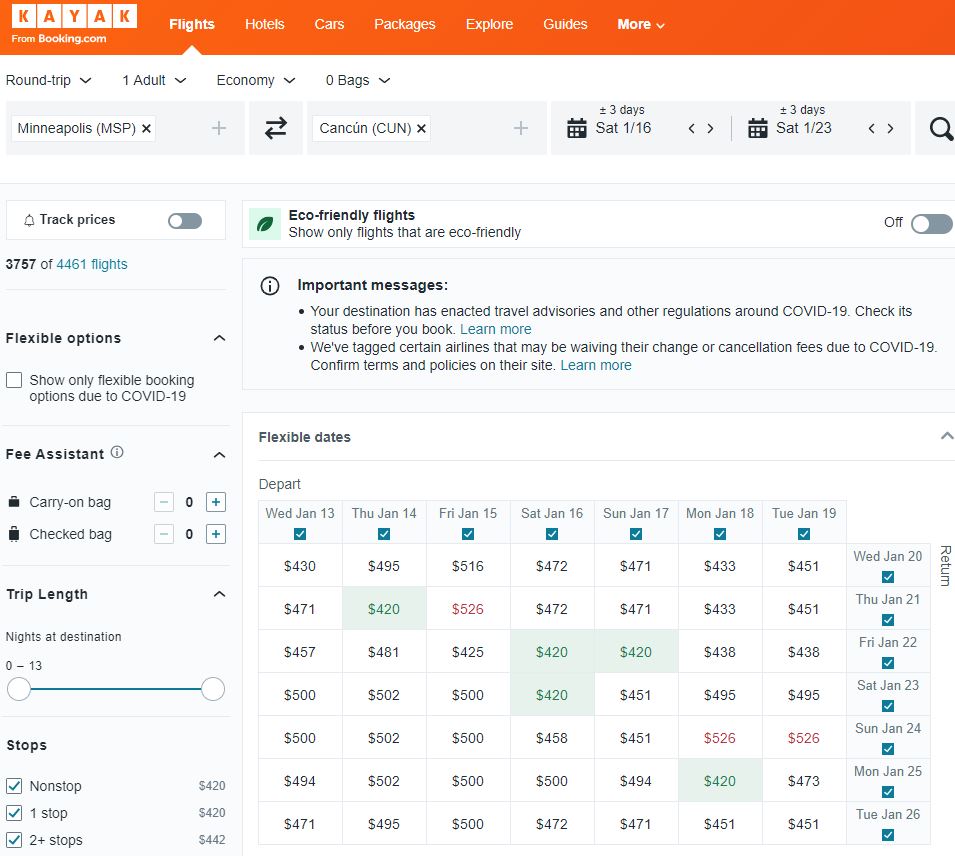**Detailed Caption:**

This screenshot shows the user interface of a website where one can book travel arrangements, specifically through the Kayak platform by Booking.com. At the top, a prominent orange-red navigation bar features the title "kayak from booking.com." 

The navigation menu includes tabs for 'Flights,' 'Hotels,' 'Cars,' 'Packages,' 'Explore,' 'Guides,' and a 'More' button for additional options. The 'Flights' tab is currently selected. The user has chosen a round trip for one adult in the economy class with no bags. 

The travel itinerary entered is from Minneapolis to Cancun for a duration of three days. On the bottom left side of the interface, an option to 'Track prices' is available, featuring a toggle switch. Below this, it states that the search has returned 3,757 of 4,461 available flights.

Additional options include the choice of eco-friendly flights, which are denoted by a small green icon. An 'Important Messages' section displays several noteworthy notifications underneath it. Flexible options are present on the left side, such as 'Fee Assistant,' 'Trip Length,' various stop options ('Non-stop,' 'One Stop,' and 'Two or more stops'), and flexible date selections, accompanied by a range of price options for different departure and return days.